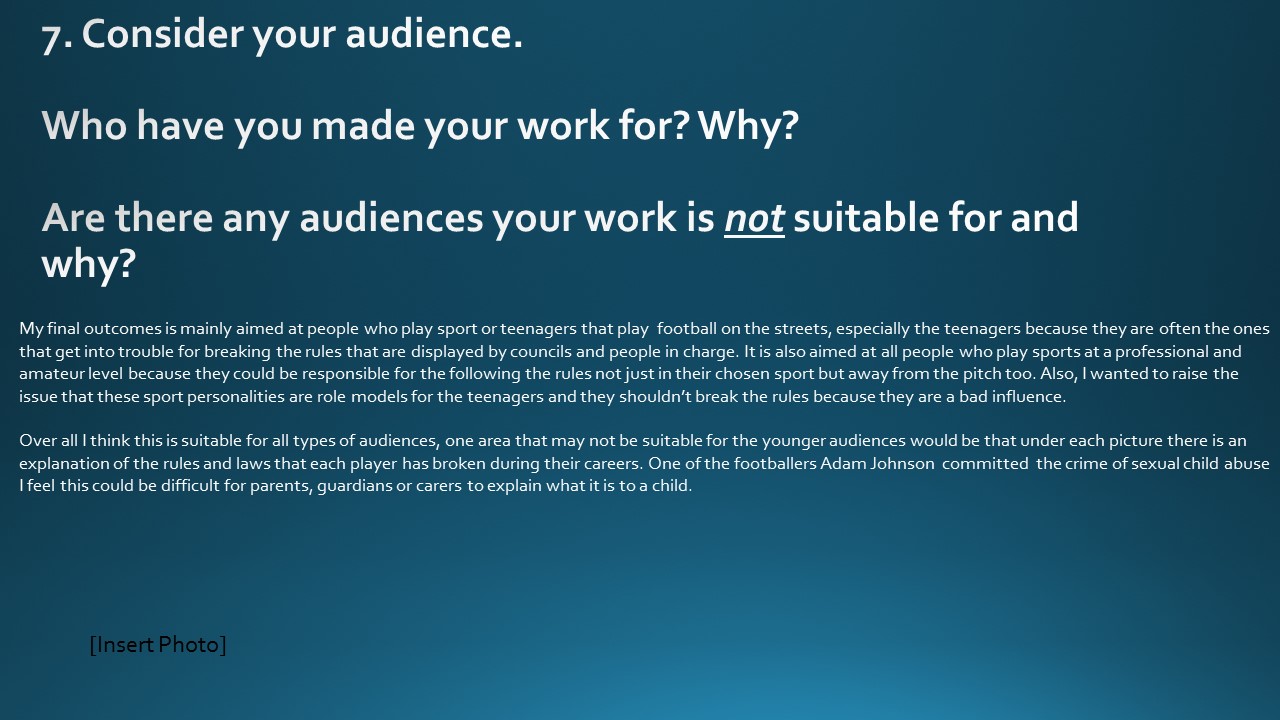The image is a slide from a PowerPoint presentation with a gradient background transitioning from dark blue-gray at the top to a lighter, almost white hue at the bottom. The white text prominently displays "7. Consider your audience" at the top left. Below this, larger text poses the questions: "Who have you made your work for? Why?" and "Are there any audiences your work is *not* suitable for and why?" with "not" italicized and underlined.

Beneath these questions, two paragraphs of smaller white text elaborate on the target audiences and potential exclusions. The content mentions that the final outcome is mainly aimed at teenagers who play sports, particularly football, on the streets. The document highlights the societal issues these teenagers face, especially from authorities, and seeks to address the behavior of professional and amateur sportspeople, suggesting they should follow rules both on and off the pitch as they are role models for young athletes.

Special attention is drawn to certain content that might be unsuitable for younger audiences, such as explicit descriptions of legal infractions by athletes, including a mention of footballer Adam Johnson’s conviction for sexual child abuse. This sensitive information could pose challenges for guardians needing to explain it to children. At the bottom left, black text in parentheses reads "insert photo," indicating a placeholder for an image.

The slide's detailed structure and content focus on preparing the reader to think critically about their audience and the appropriateness of their material for different groups.